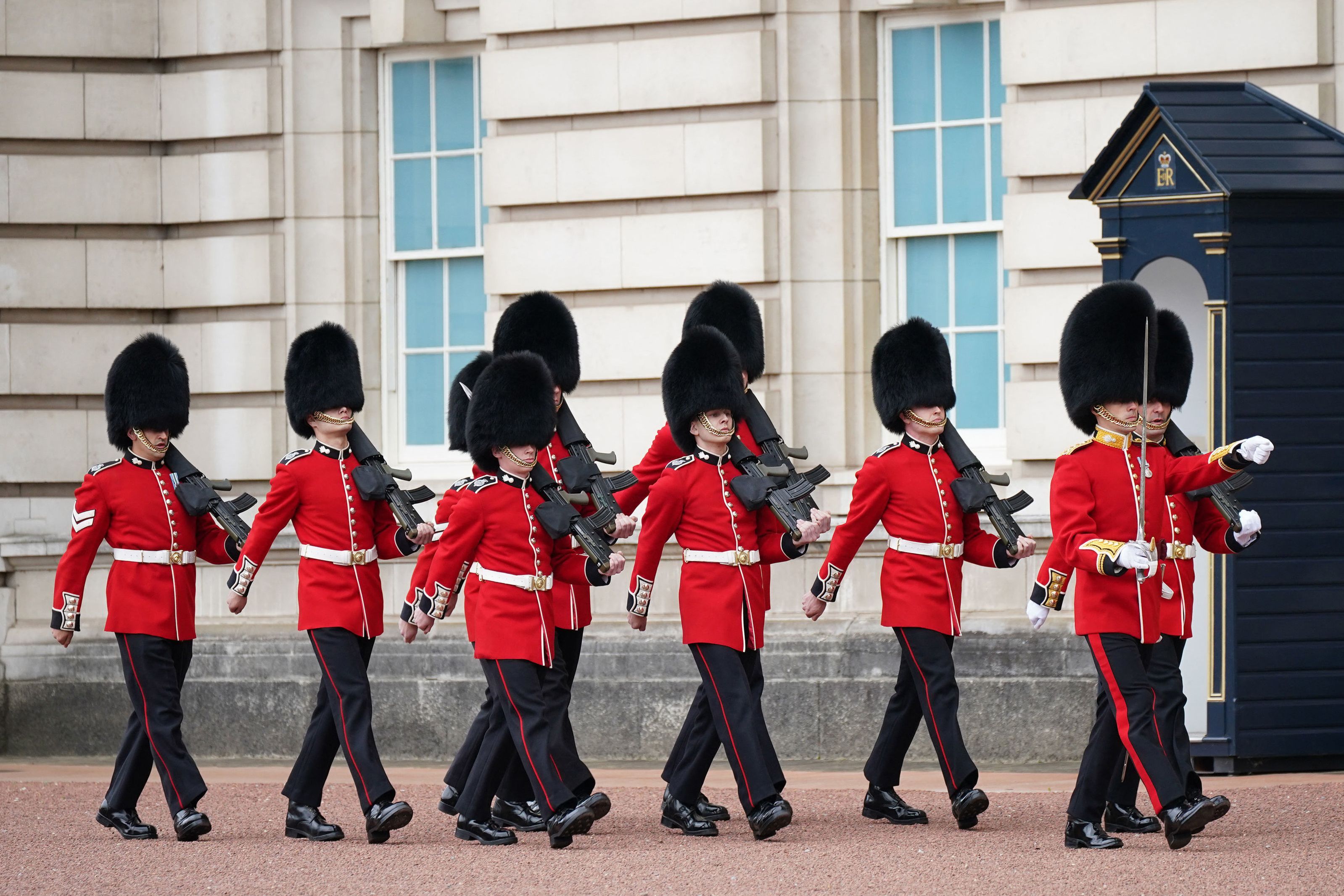The vertical rectangular image depicts a group of Royal Guards marching in front of Buckingham Palace. The guards are dressed in traditional uniforms consisting of tall, black fuzzy hats, red jackets with white belts, black pants accented with a red stripe, and black leather shoes. Among the soldiers, all but the leading guard are carrying long black rifles over their left shoulders, while the leader wields a silver sword in his right hand. They are positioned in front of the white exterior of the palace, which features two rectangular windows with white trim and opaque glass. To the far right of the image, there is a dark blue triangular-roofed guard post. The ground beneath them has a brick-like appearance, adding texture to the scene. This photograph effectively captures the disciplined and iconic nature of the Royal Guard in their ceremonial duties.